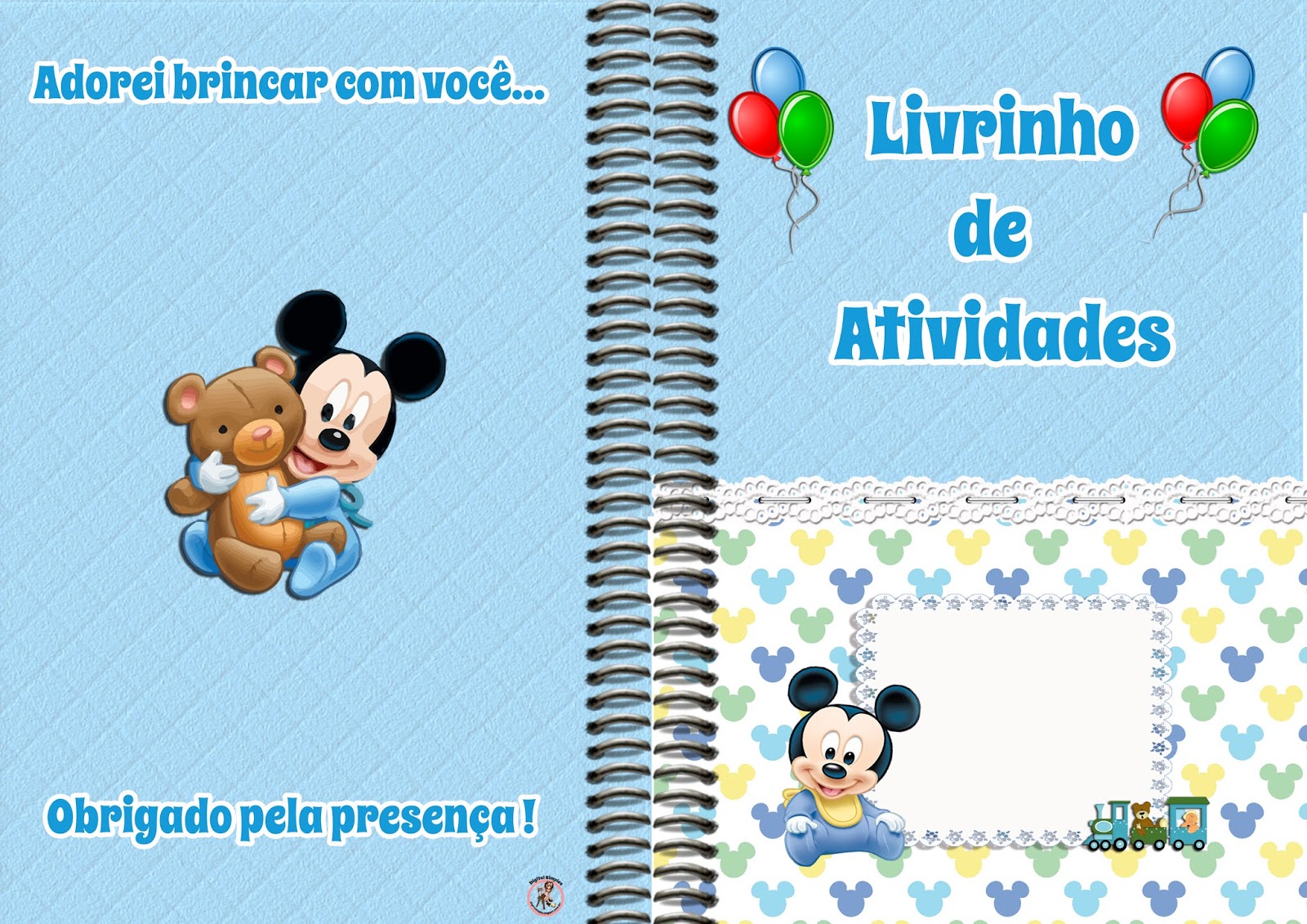This image is a detailed drawing resembling an open spiral-bound baby journal with a soft, baby blue background featuring a quilted pattern. The left page, which appears to be the back cover, shows baby Mickey Mouse in a blue onesie snuggling up with a teddy bear in the center. Above and below Mickey, there are words written in Portuguese, “Adore Brincar Com Voce” and “Obrigado Pela Presencia”. The right page, representing the front cover, features the title "Livrinho de Atividades" at the top, with colorful clipart balloons in red, green, and blue flanking the text. Additional decorative elements include scattered Mickey Mouse ears and a little toy train at the bottom right. Near the bottom of this page is a rectangle, perhaps a designated space for a baby photo, adorned with another baby Mickey wearing a bib, and a small clipart train at the lower corner. The booklet overall gives off a playful, inviting air, perfect for a baby’s activity or memory book. Behind the graphics, subtle outlines of Mickey Mouse heads in varying shades of blue, green, and yellow add extra charm to the design.